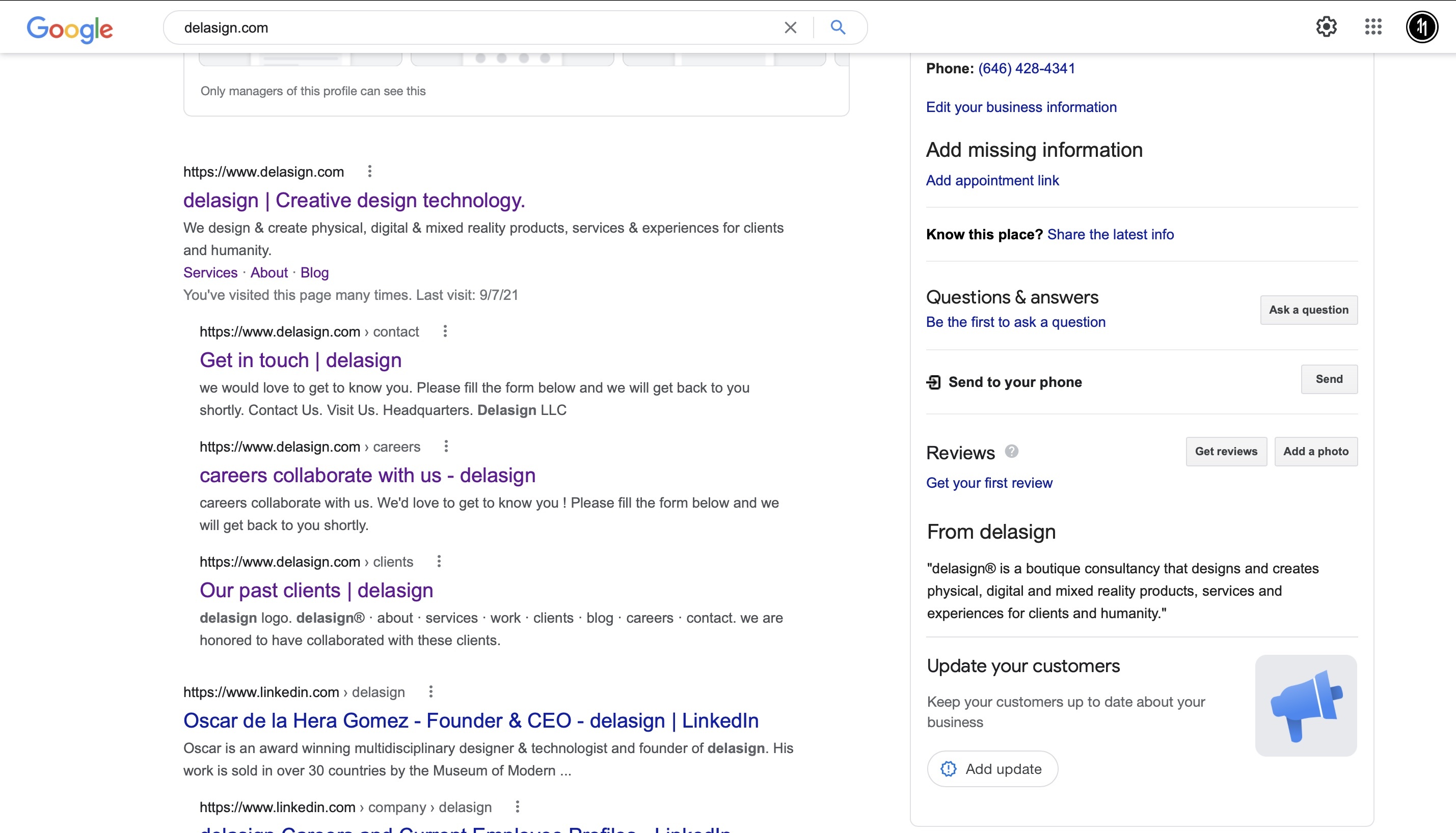The screenshot displays a Google search results page from a computer. In the upper left corner, the recognizable Google logo is visible, featuring the familiar rainbow-colored letters. To the right of the logo, the search bar shows the query "DeLaSign.com."

Below the search bar, several search results related to DeLaSign.com are listed. The first result is prominently displayed with the title "DeLaSign - Creative Design Technology" in purple text. It is followed by a description stating, "We design and create physical, digital, and mixed reality products, services, and experiences for clients and humanity." Below the title, clickable options in purple text are available, such as "Services," "About," and "Blog." An additional note underneath indicates that the user has visited this page multiple times, with the last visit recorded on September 7, 2021.

Further, the search result includes a "Get in touch" link in purple text, encouraging users to fill out a form to be contacted by DeLaSign. On the right side of the page, there is a section that highlights a phone number in blue, along with other useful options like "Add missing information," "Add appointment link," "Questions and answers," "Send to your phone," and "Reviews." 

At the bottom right corner of the screenshot, a small blue megaphone icon is visible, indicating additional features or announcements. 

Overall, this screenshot captures a comprehensive view of the Google search results page for DeLaSign.com, showcasing the various interactive elements and detailed information about the consultancy's offerings.